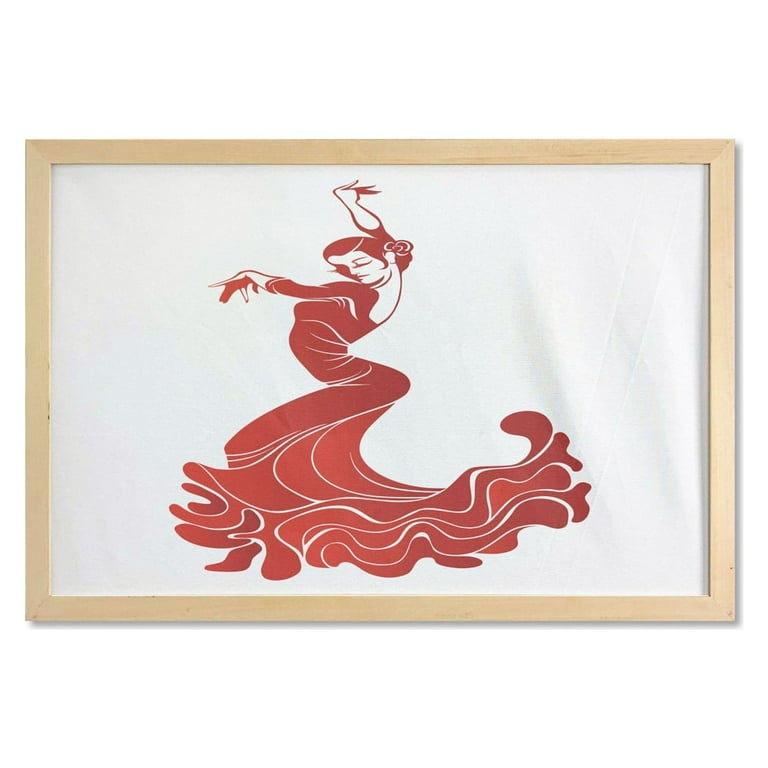The image portrays an artwork depicted within a light wooden frame. The artwork itself features a white canvas or fabric background, notably appearing slightly wavy on the right side, suggesting it isn't tightly stretched. Dominating the center is a cartoon-style figure of a woman in an exaggerated dancing pose. She is adorned in a long, flowing red dress with an undulating bottom that mimics ocean waves. Her body features, particularly her hips and waistline, are highly exaggerated, enhancing the cartoon-like essence. The woman is engaged in a dynamic dance move, likely salsa, with her arms raised elegantly in the air, her head tilted back, and her eyes closed, exuding a sultry, joyful expression. Her hair is pulled back, accentuated by a flower tucked into it. The minimalistic background and absence of surrounding elements imply a product image focus on the artwork alone.